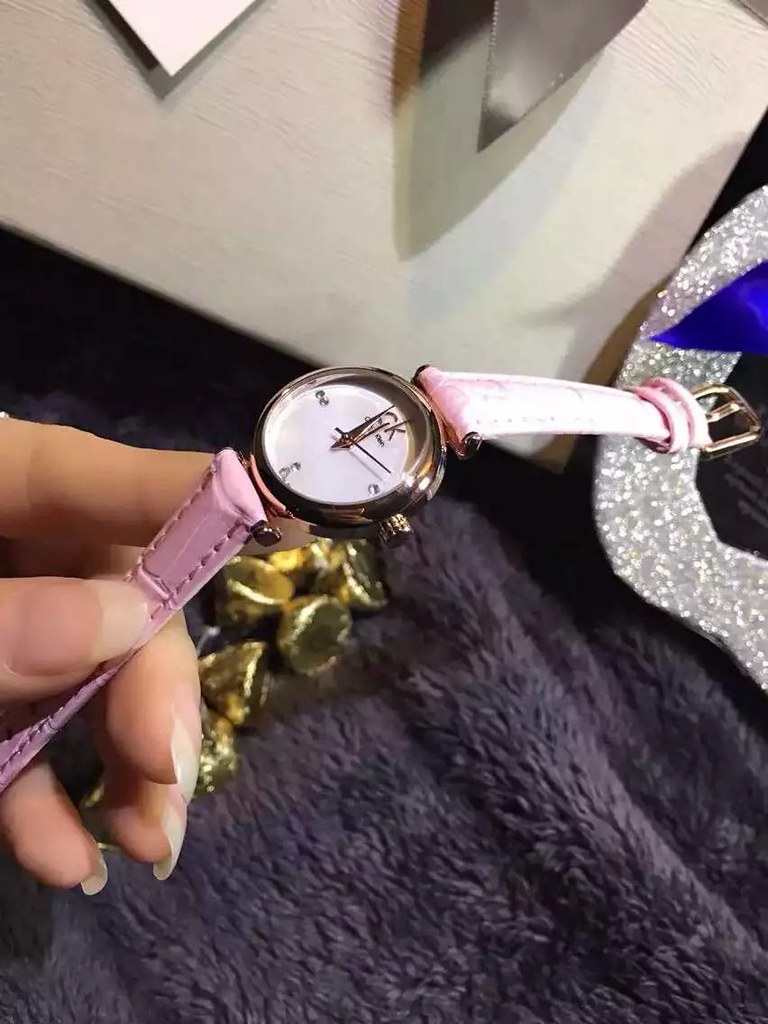In the image, a well-manicured woman with relatively long fingernails is holding a minimalist Calvin Klein watch. The watch features a thin pink leather strap and a gold casing around the crown. It has small diamonds marking the positions of 12, 3, 6, and 9 on the watch face, which adds a subtle touch of elegance. The watch is fastened with a clasp. The scene is set against a backdrop of a shaggy purple blanket and a white wall adorned with a silver-framed picture. Additionally, a small blue and silver object can be glimpsed at the bottom of the frame, though its purpose remains unclear.